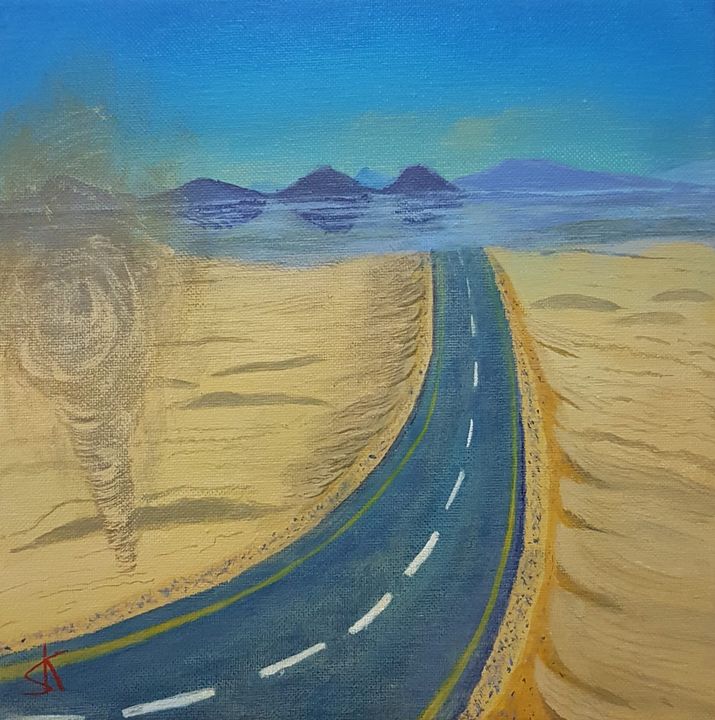The painting depicts a two-lane paved road that begins in the bottom left corner and curves into a straight path as it progresses towards the center of the image, eventually disappearing at the horizon. The road, marked with a white dotted line in the middle and yellow lines on the sides, traverses through a sandy or desert-like landscape. The sand is a light yellowy tan color, and a small dust devil or sand tornado is visible on the left side of the road. In the background, a range of blue mountains stretches beneath a bright blue sky. The painting is signed "SK" in red in the bottom left corner. The artwork has an amateurish quality, lacking photorealistic details, and the road itself seems to have a bluish tint.